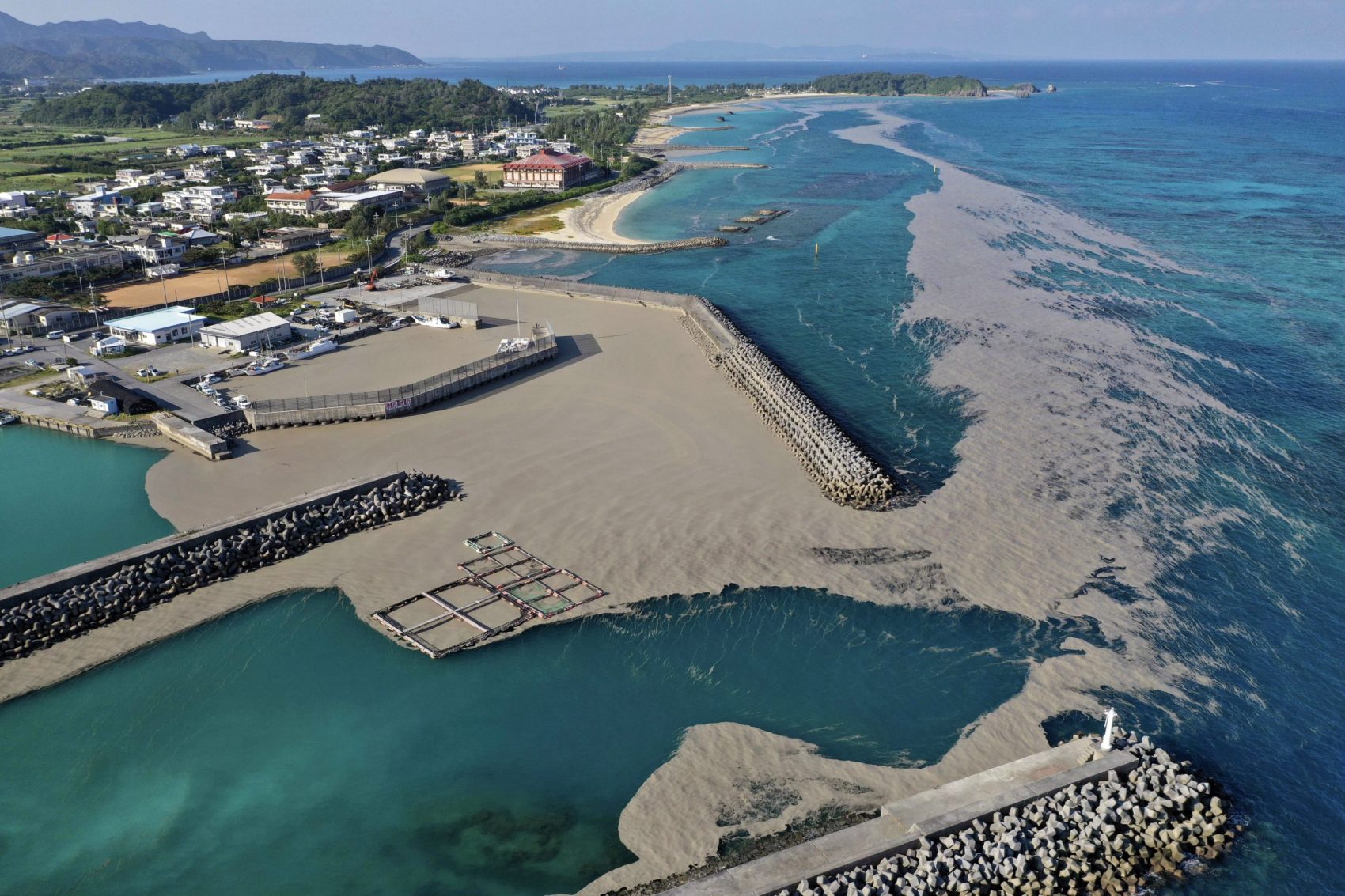This aerial photograph captures a vivid scene of a clear, blue-green coastal area, featuring a multifaceted harbor along a picturesque coastline. The coastline is lined with vibrant, rolling green hills and distant mountains that paint a serene backdrop. A series of breakwaters or jetties angle themselves prominently, creating protected sections of the harbor, which are dotted with residential buildings varying from dark gray to white, with occasional red and blue structures standing out. The water, exceptionally clear and shallow, exhibits swirls of unusual flat gray foam, contrasting against the natural scenery. Sand curves along the shore, leading to dark beaches. An airport sits closely adjacent to the water, emphasizing the blend of natural beauty and infrastructural development. Floating structures resembling lines of cages atop the water indicate some form of marine activity, adding to the richness of the scene. Farther back, additional islands and mountainous outlines frame the expansive and tranquil ocean views under a sky transitioning to a light blue hue.